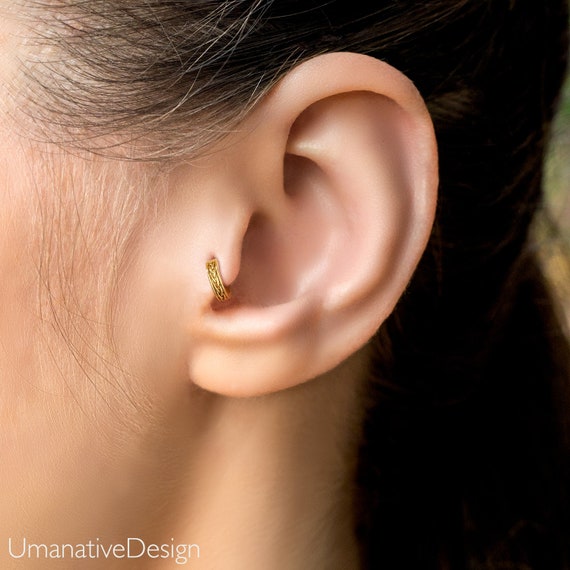The image is a close-up shot of a human ear, which appears to belong to a female. The ear is petite and delicate, with a single piercing located on the inner part, near the sideburns. Adorning the piercing is an intricately designed gold band earring. The ear is not adorned with any other piercings. The individual has greyish hair around the sides, while the rest of the hair is dark and flows down the back in a long style. At the bottom of the image, the logo "Humanitive Design" is prominently displayed.